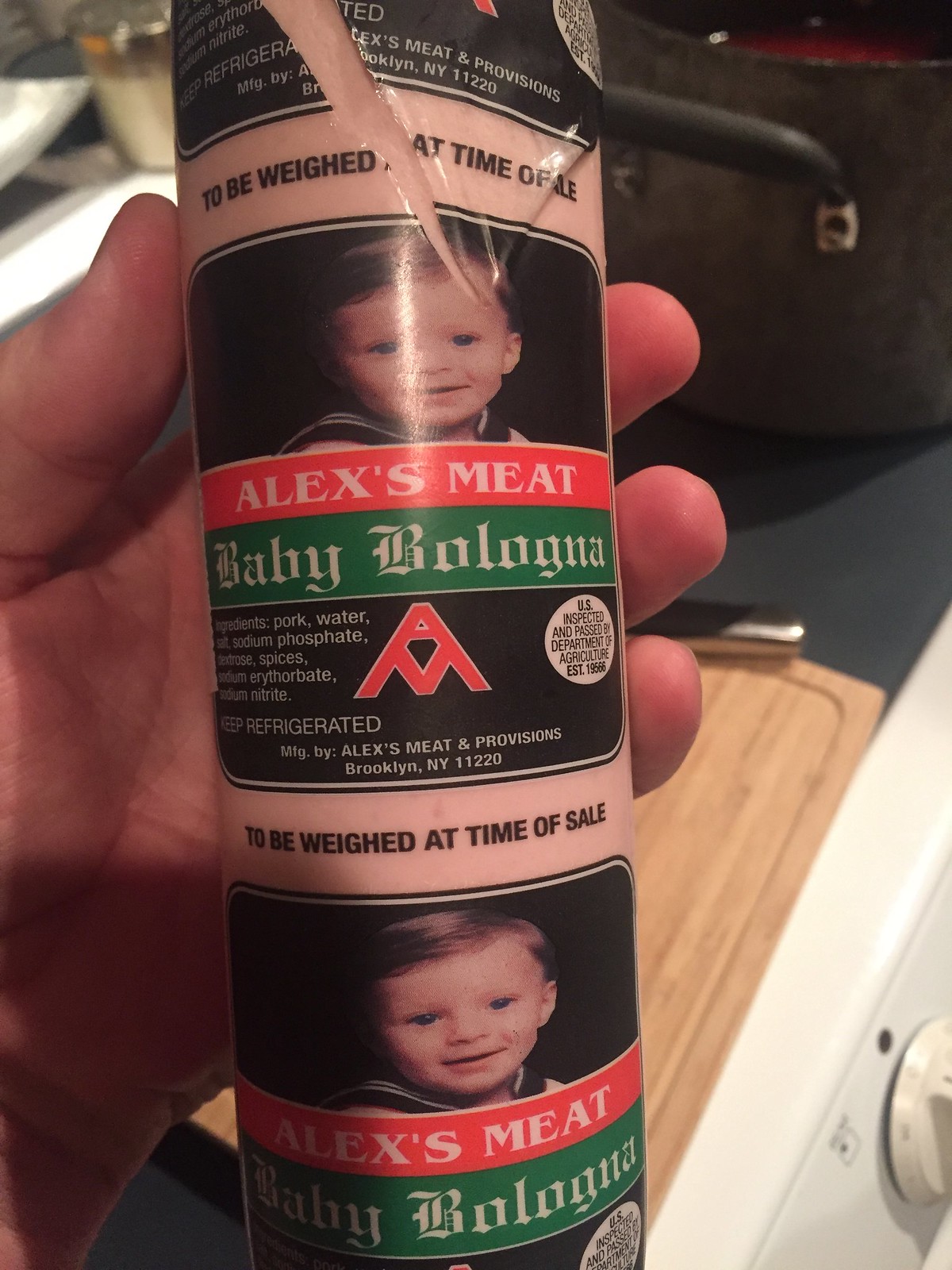In the image, a person is holding up a package of food in their left hand, prominently displaying it towards the camera in what appears to be their home kitchen. The package, partially split open, reveals a roll or tube of Baby Bologna made by Alex's Meat and Provisions. The label on the packaging is rich in detail: the top portion shows a photograph of a young, dark-haired child, approximately three or four years old, dressed in a blue sailor-type uniform with white stripes. Below the image, the brand name "Alex's Meat" is boldly printed in white text against a red horizontal rectangle, and beneath that, "Baby Bologna" is inscribed in stylized white text on a green rectangle. Additional information on the label includes a list of ingredients, such as pork and sodium phosphate, and a clear instruction to keep the product refrigerated. The background of the kitchen includes a cast iron cooking pot with a black handle, a wooden chopping board with ridges, and an off-white appliance with a handle dial on the bottom right. The meticulously organized kitchen backdrop underscores the domestic setting of this detailed and homely capture.